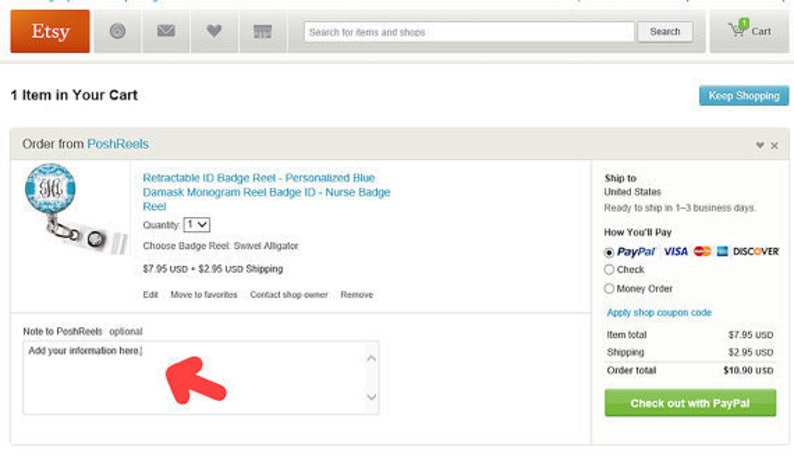The image is a screenshot from an Etsy webpage showcasing a product listing. In the upper left-hand corner, there's a deep orange-red box with "Etsy" prominently displayed in white print. Moving horizontally from this box, there are various icons including a clickable heart, and other functional links. A search bar labeled "Search for items and shops" is positioned at the top, accompanied by a search option. Adjacent to this is a shopping cart icon with a green indicator showing the number "1," signifying one item in the cart.

Below the horizontal navigation bar, the text states "One item in your cart" in black print, referencing an order from "Posh Reels". The product description reads "Retractable ID badge reel - Personalized blue Damask monogram reel badge ID - Nurse badge reel," priced at $7.95 USD with an additional shipping cost of $2.95 USD. A red arrow, drawn on the page, points to the lower left-hand area where it instructs "Add your information here." Further details on the page indicate that the item ships to the United States and the payment method is via PayPal, with a green "Check out with PayPal" button readily available for completing the purchase.